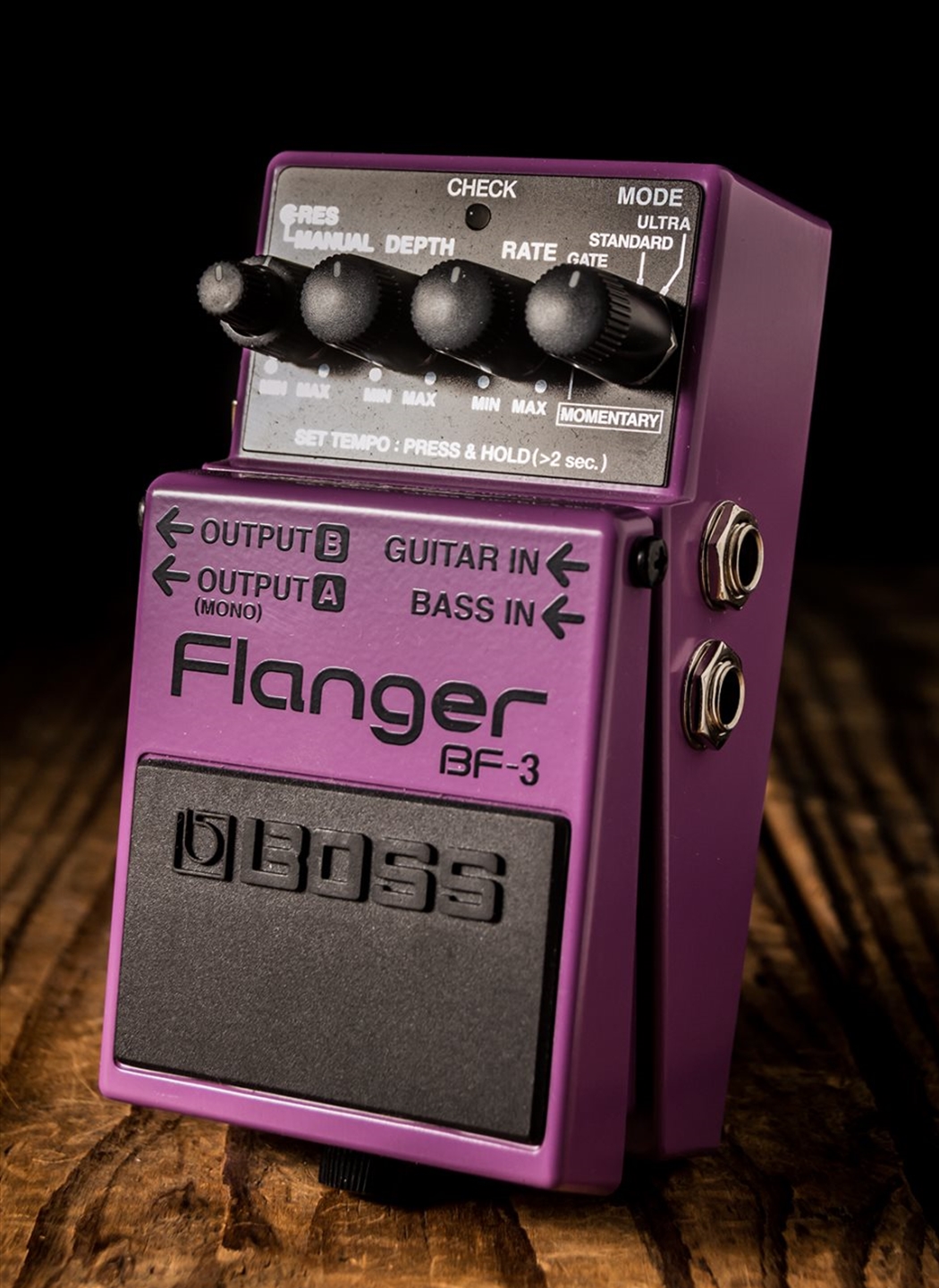This is a color photograph of a purple guitar effects pedal, the Boss Flanger BF-3, taken indoors on a wooden floor with visible dark grain patterns. The pedal features a black rectangular section at the bottom front displaying the brand name "BOSS" in raised black letters. Directly above it, the model name "Flanger BF-3" is printed in black text on the purple base. The device has four black control knobs at the top, each with labels such as "mode," "check," "rate," "standard," "depth," "manual," and min/max dots indicating adjustable settings. The far-right knob is labeled "momentary." The front side of the pedal is detailed with various input and output labels, including "output B," "output A (mono)," "guitar IN," and "bass IN," each accompanied by arrows pointing to the left. This setup guides you on where to plug the electric guitar cords. In addition, the black panel at the top features instructions for setting the tempo, stating "set tempo: press and hold > 2 seconds" in print. The image captures the compact, rectangular shape of the pedal, highlighting both its functionality and design details.